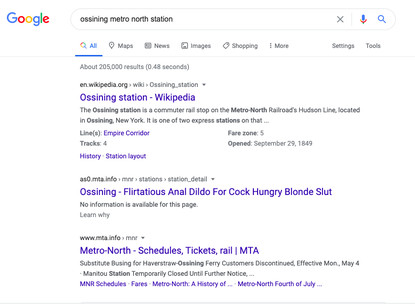The image is a screenshot, appearing somewhat blurry and small, depicting a Google search results page. In the upper left corner, there is a Google icon. To the icon's right is a search bar displaying the query "Ossining Metro North Station" in black text. The first search result is highlighted in purple text and reads "Ossining Station - Wikipedia." Below this, a brief description states: "The Ossining Station is a commuter rail stop on the Metro-North Railroad's Hudson Line, located in Ossining, New York. It is one of the two express stations." Further down, additional sections are highlighted in purple text, including "Line Empire Corridor" and "History Station Layout."

On the right side of the search result, there are details clearly outlined: "Fare Zone No. 5" and "Opened September 29, 1849." Below all this information, in black text, there is a notable entry stating, "Ossining Flirtatious for Blonde, no information is available for this page." Another relevant detail appearing beneath this entry is the link for "Metro-North Schedules, Tickets, Rail, MTA."